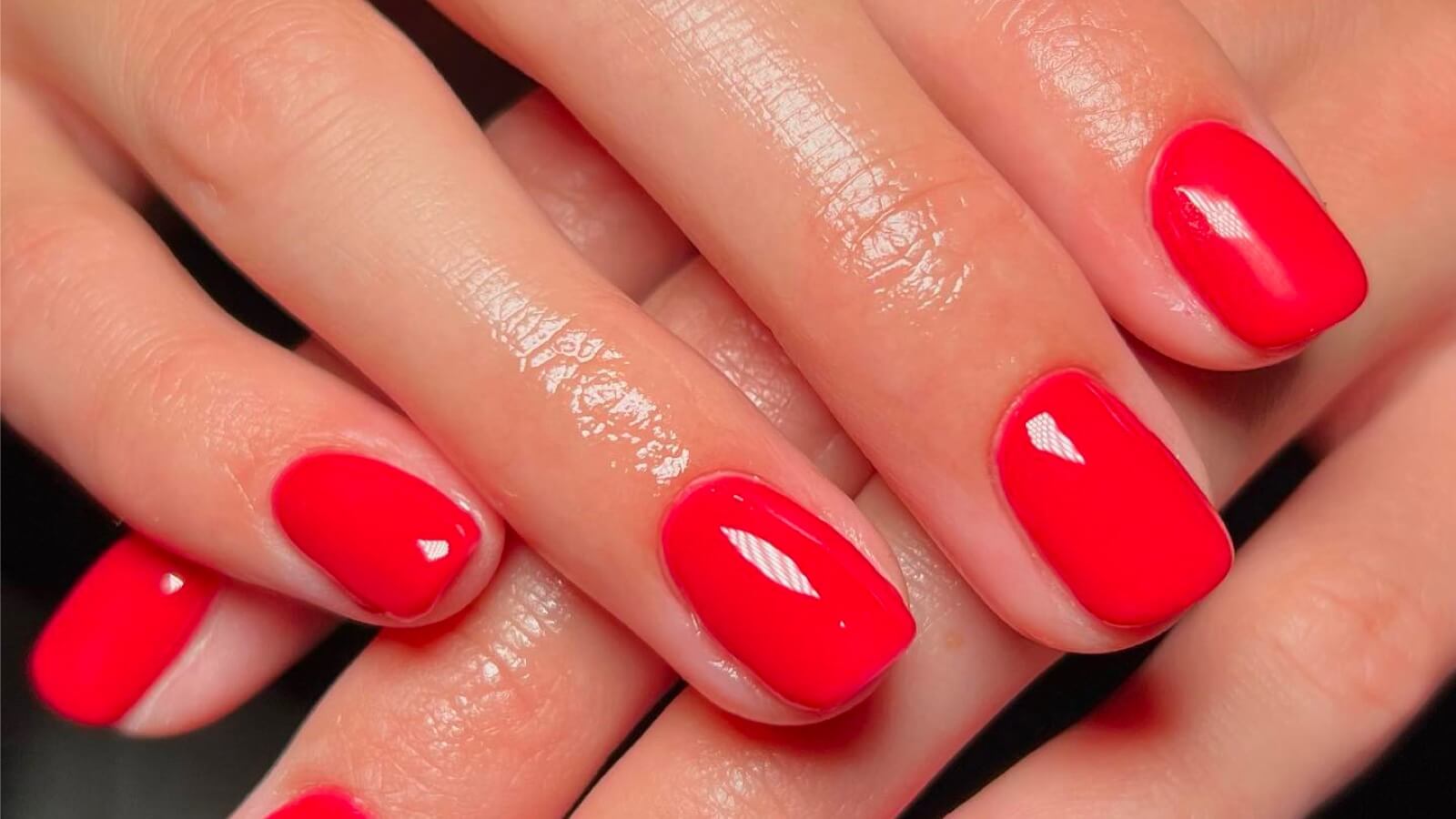This close-up image features two hands, likely of a Caucasian woman, layered atop each other against a dark, possibly black, background. The hands are positioned cross-hatched, with the left hand entering from the upper right corner diagonally down and to the left, and the right hand entering from the upper left corner diagonally down and to the right, resting over the other hand's fingers. Both hands exhibit glossy, shiny skin, giving the impression they have been recently oiled. The nails are painted a vibrant fire-engine red, with a thick layer of polish reflecting white highlights where the light catches. The upper hand displays all its nails clearly, while only two fingernails of the lower hand are visible due to the cropping of the image. The nails are uniformly cut short and rounded at the ends. The picture, highly detailed, also showcases the texture and lines of the skin, emphasizing the wet, glossy look.